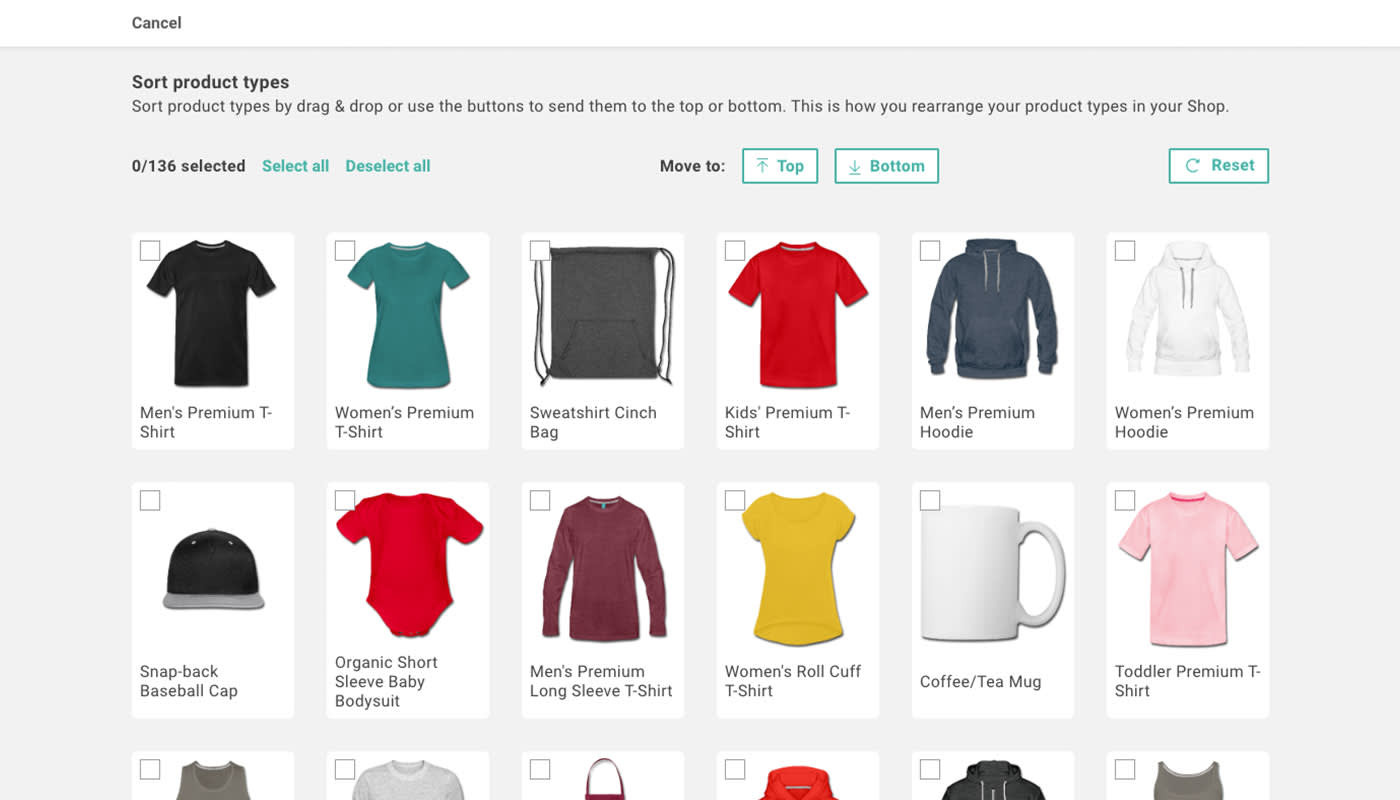In the background of this light gray interface, someone appears to be engaged in setting up an online clothing store. The screen displays a banner with the option to “Cancel” operations, followed by instructions in black text: "Sort prototypes by drag and drop or use the buttons to send them to the top or bottom." This feature allows the user to rearrange the prototypes within their shop. Below these instructions, there’s a display reading "0 / 136 selected," accompanied by green buttons labeled "Select All" and "Deselect All."

Further down, in black text, it reads "Move to...," with two outlined green boxes labeled "Top" and "Bottom" for easy placement of prototypes. A similar green-outlined box to the right reads "Reset."

The interface organizes items into rows of six per line. The first row includes:
1. Men's Premium T-Shirt (Black)
2. Women's Premium T-Shirt (Green)
3. Sweatshirt (Light Gray)
4. Drawstring Bag (Light Gray)
5. Kids’ Premium T-Shirt (Red)
6. Men's Premium Hoodie (Gray)

In the second row, the items listed are:
1. Women's Premium Hoodie (White)
2. Snapback Baseball Cap (Black)
3. Organic Short Sleeve Baby Bodysuit (Red)
4. Men's Premium Long Sleeve T-Shirt (Red)
5. Women's Rose Cut T-Shirt (Yellow)
6. Coffee/Tea Mug (White)
7. Toddler Premium T-Shirt (Light Red)